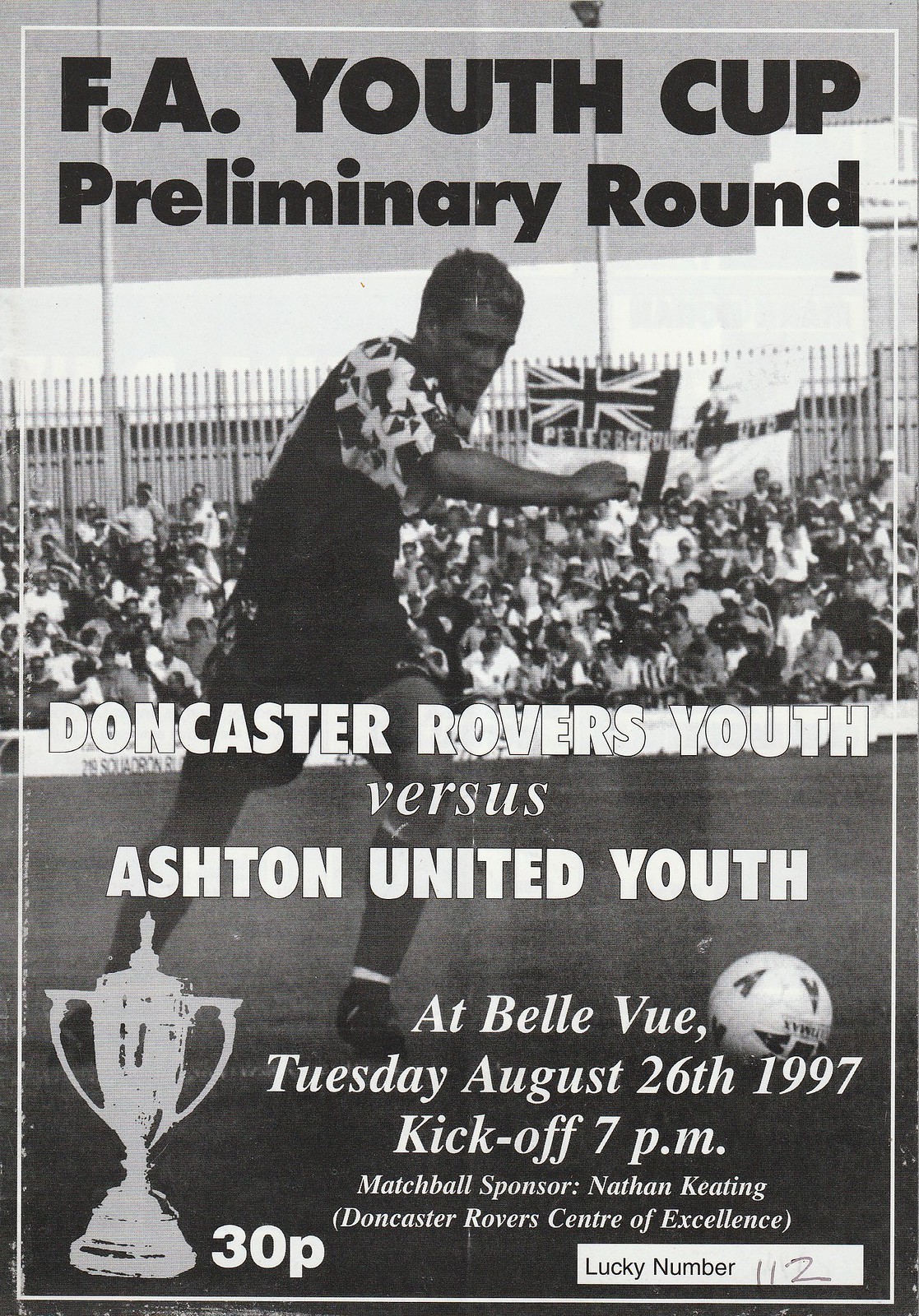This black and white poster advertises the FA Youth Cup Preliminary Round, featuring Doncaster Rovers Youth versus Ashton United Youth. The event is scheduled to take place at Bellevue on Tuesday, August 26, 1997, with kickoff at 7 p.m. The poster highlights the match ball sponsor, Nathan Keating from Doncaster Rovers Center of Excellence, and includes a lucky number 112. An image on the poster shows a soccer player mid-action, possibly about to kick the ball, with a large crowd of spectators seated in bleachers in the background. A British flag is being raised among the crowd. For additional detail, a two-handled trophy icon is displayed on the bottom left corner, next to the price mark of 30p. The player depicted is wearing a black uniform, and there's a railing behind the crowd for safety.